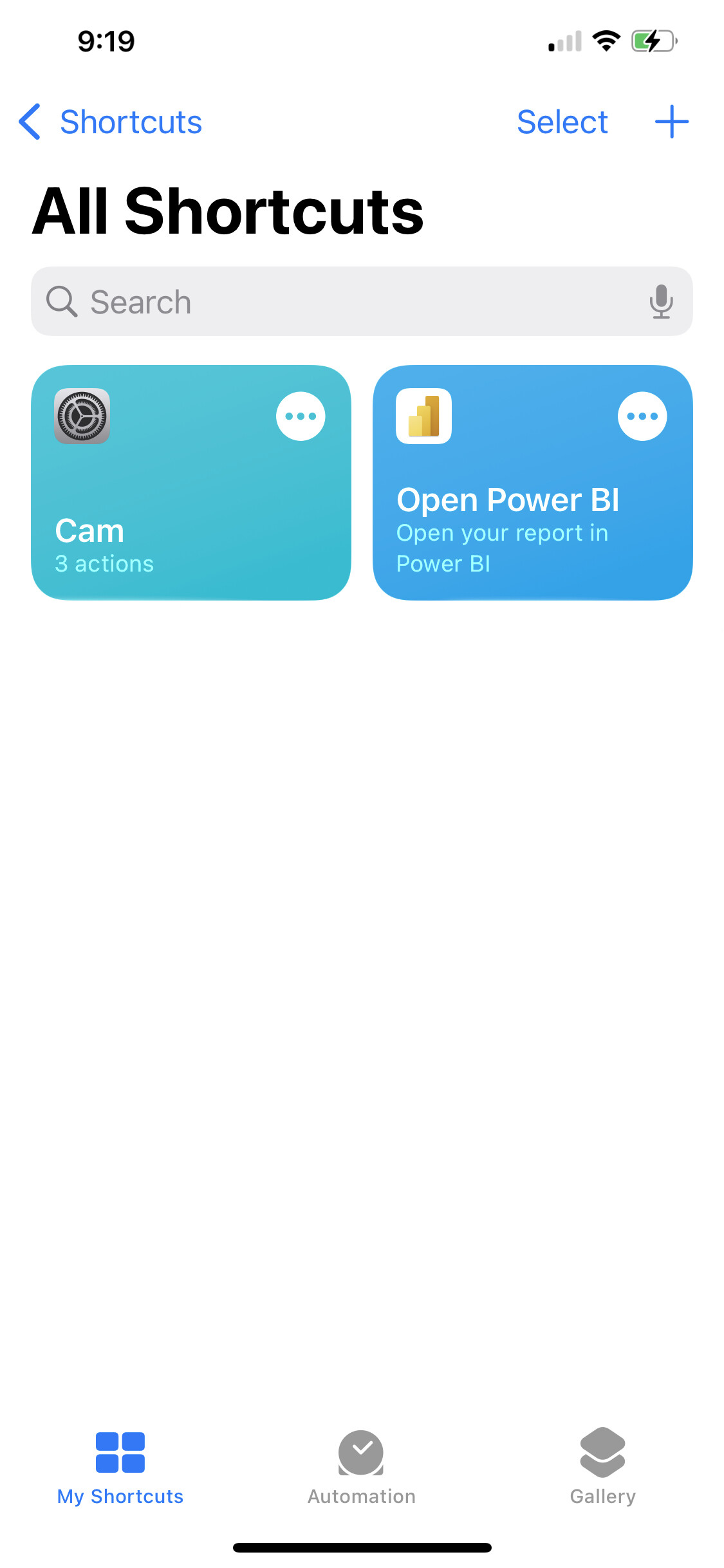The image displays a smartphone screen with detailed information and multiple icons. The phone's battery life is below 50%, indicated by a partially filled green bar on the left side, transitioning to white on the right side. The connection strength shows one out of four bars filled, indicating limited connectivity. The time displayed is 9:19 AM, with the word "Shortcuts" written beneath it in light blue and an arrow pointing to the left.

Below the battery icon, the word "Select," written in blue and accompanied by a plus sign, is visible. In large black font, the text "All Shortcuts" is prominently displayed beneath that section, followed by a light gray search bar featuring a microphone icon on the right.

The interface includes two rounded square icons:
- The first icon on the left is teal and has a settings icon on the left side, along with a white circle containing three dots on the right side. Below this icon, the text "CAM" is written, accompanied by the phrase "3 actions."
- The second icon on the right prompts, "Open Power BI," directing users to open a report in Power BI. This icon features a graphic resembling bar charts and a circle with three dots inside it.

At the bottom of the screen, three tabs are visible: "My Shortcuts," "Automation," and "Gallery."